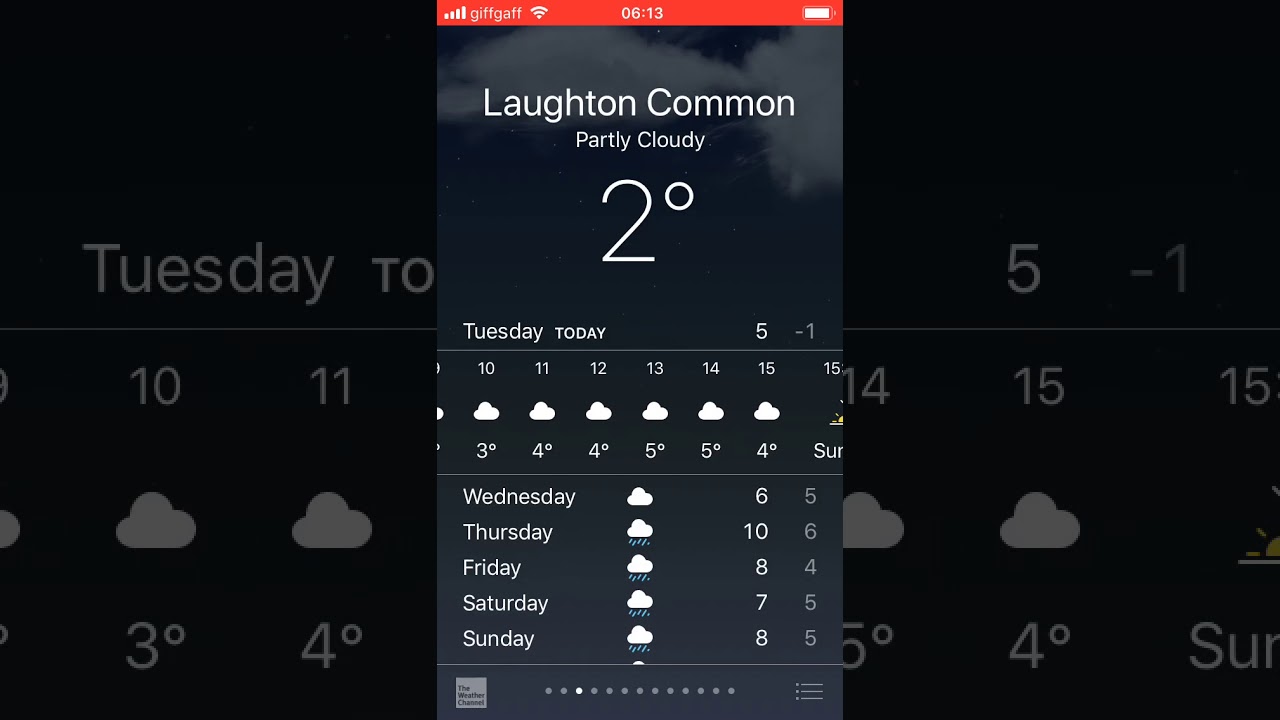The image depicts a smartphone screen displaying a weather app. At the top, there's a red horizontal status bar showing full cellular signal strength with four bars and the carrier name "GIFGAF". Adjacent to it, the Wi-Fi icon also shows four bars, indicating strong connectivity. The time displayed is 6:13, and on the far right, there's an icon indicating a fully charged battery.

Below the status bar, the weather app interface is visible. The main section at the top indicates the current weather condition, described as "Partly Cloudy" with a temperature of 2 degrees Celsius. It's a Tuesday, and the forecast for today includes a high of 5 degrees and a low of -1 degree.

The forecast breakdown for the day shows hourly conditions from 10:00 to 15:00, each hour marked with a cloudy icon:
- 10:00 - 3 degrees Celsius
- 11:00 - 4 degrees Celsius
- 12:00 - 4 degrees Celsius
- 13:00 - 5 degrees Celsius
- 14:00 - 5 degrees Celsius
- 15:00 - 4 degrees Celsius

Below the hourly breakdown, the weather forecast for the next few days is provided, each with corresponding icons and temperature ranges:
- Wednesday: Cloudy, high of 6 degrees, low of 5 degrees
- Thursday: Cloud with rain, high of 10 degrees, low of 6 degrees
- Friday: Cloud with rain, high of 8 degrees, low of 4 degrees
- Saturday: Cloud with rain, high of 7 degrees, low of 5 degrees
- Sunday: Cloud with rain, high of 8 degrees, low of 5 degrees

The weather information is sourced from The Weather Channel, presented within a larger image of the weather app.